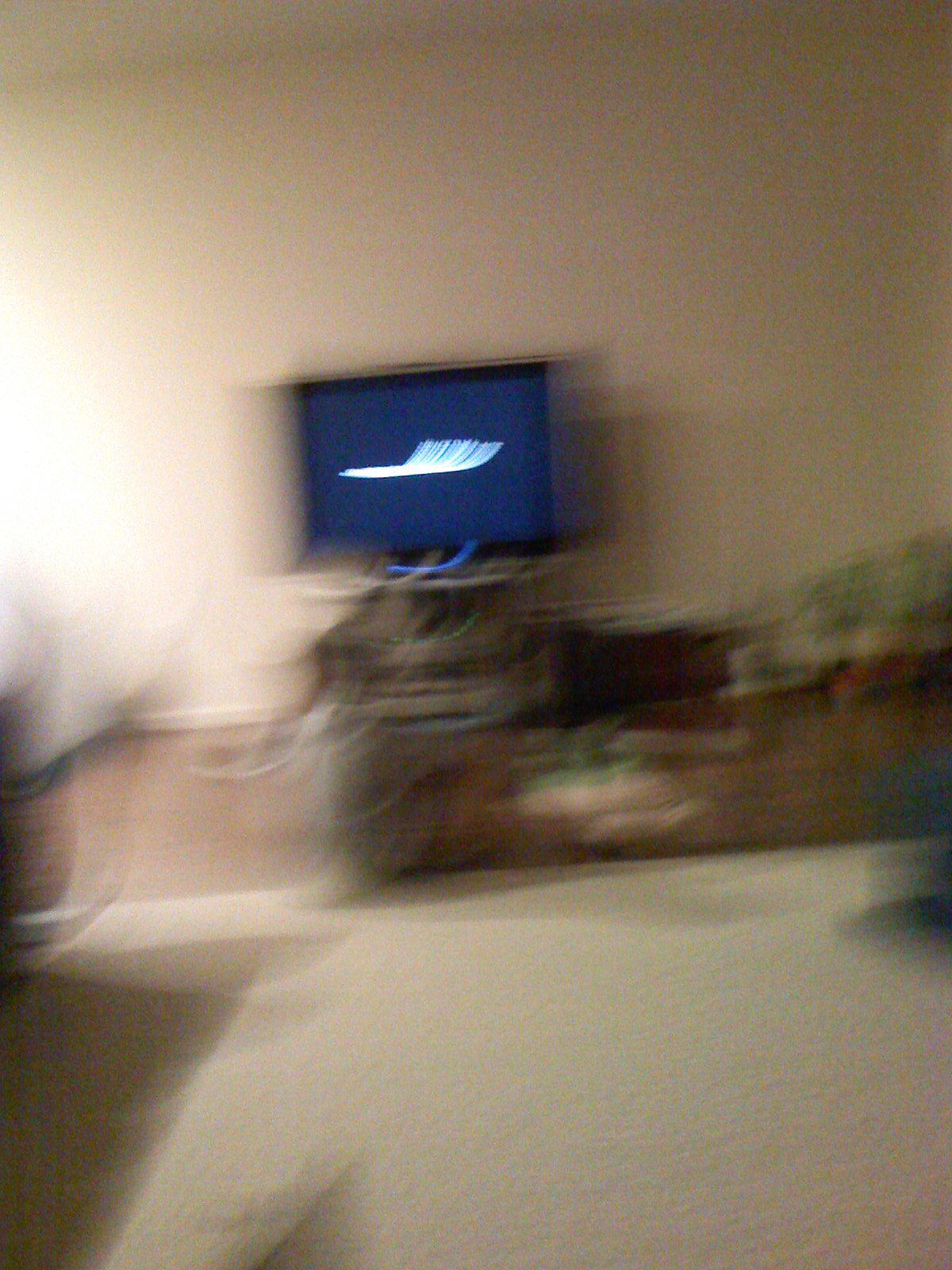The image depicts a very blurry and out-of-focus photograph of a small television up against an off-white or light brown wall. The TV screen displays a dark blue background with white lettering and a feather-like swoosh of white light. The TV appears to be on a piece of furniture, potentially a stand or credenza, with a brown or wooden top. The room seems to be an interior space, possibly a living room, featuring cream-colored carpet covering most of the floor but cropped out to the left and right. The photograph is so blurred that it seems to have been taken while in motion, making the surrounding objects indistinguishable. Hints of tan, brown, light green, and blue colors are scattered around, with a green object, possibly a plant, visible on the right side. There are shadows suggesting the presence of other furniture, and a light source is coming in from the left side of the image.